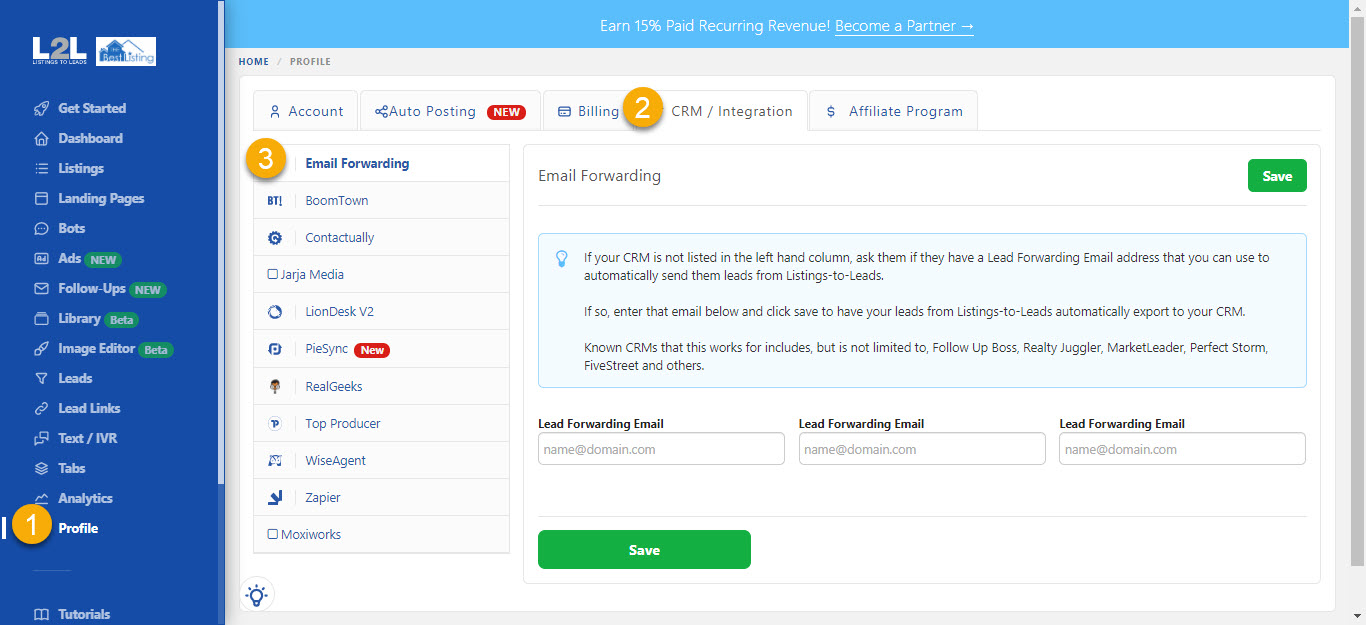This screenshot showcases the profile screen of a desktop application, providing a comprehensive guide through an organized interface. On the far left, a thick blue panel features the L2L logo at the top, with various categories listed beneath it. Notably, the last category, 'Profile,' is marked with an orange circle containing the number '1,' indicating the first step in the process.

To the right, a large white panel occupies the majority of the screen. This panel is divided into five tabs at the top: 'Account,' 'Account Posting,' 'Billing,' 'CRM Integration,' and 'Affiliate Program.' The 'CRM Integration' tab is highlighted with an orange circle marked with the number '2,' signifying the second step.

Underneath the 'CRM Integration' tab, a smaller panel titled 'Email Forwarding' appears in dark blue. This section is also indicated by an orange circle with the number '3,' representing the third and final step in the sequence.

The visuals use these numbered orange circles to guide the user through the steps: first, click on 'Profile'; second, navigate to 'CRM Integration'; and finally, select 'Email Forwarding.' The screenshot serves as an instructional aid, clearly detailing the step-by-step process within the application.